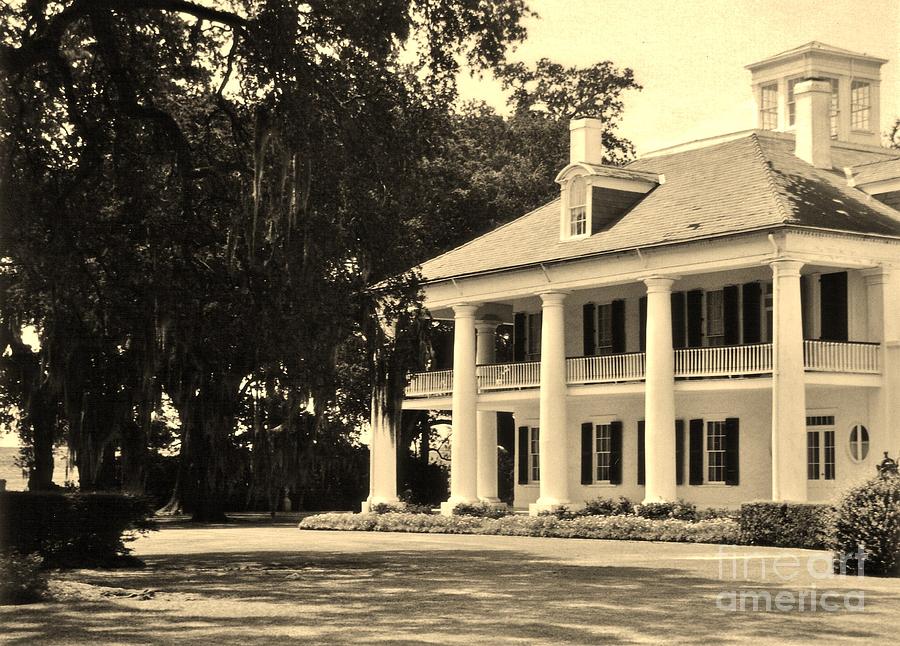This black-and-white photograph, subtly tinted with brown-yellow hues, captures an imposing two-story southern estate. The front facade features five massive Roman-style columns extending from the ground to the roof, which add an air of grandeur to the white house. The main structure boasts an angled, slanted roof with a prominent windowed gable in the center, topped by a rectangular cupola with wide windows, giving a 'crowned' appearance. The house also has vertical windows adorned with black shutters, arranged in horizontal rows across both floors.

The bottom story has an expansive porch, mirrored by an upper porch that extends the entire width of the house and wraps around the left side. These porches are fronted by low bushes, giving way to a large, meticulously maintained lawn. Interspersed around the estate are several tall trees, including what appear to be weeping willows, contributing to the grand, southern ambiance suggested by the architectural style and surrounding flora. The chimneys, one positioned to the left and one to the right of the roof, add to the balanced visual symmetry of the residence.

In the bottom right corner of the image, fine text reads "Fine Art America," subtly marking the artwork. This elegant southern home, captured in high-quality vintage style, combines classical architectural elements with a picturesque natural setting.